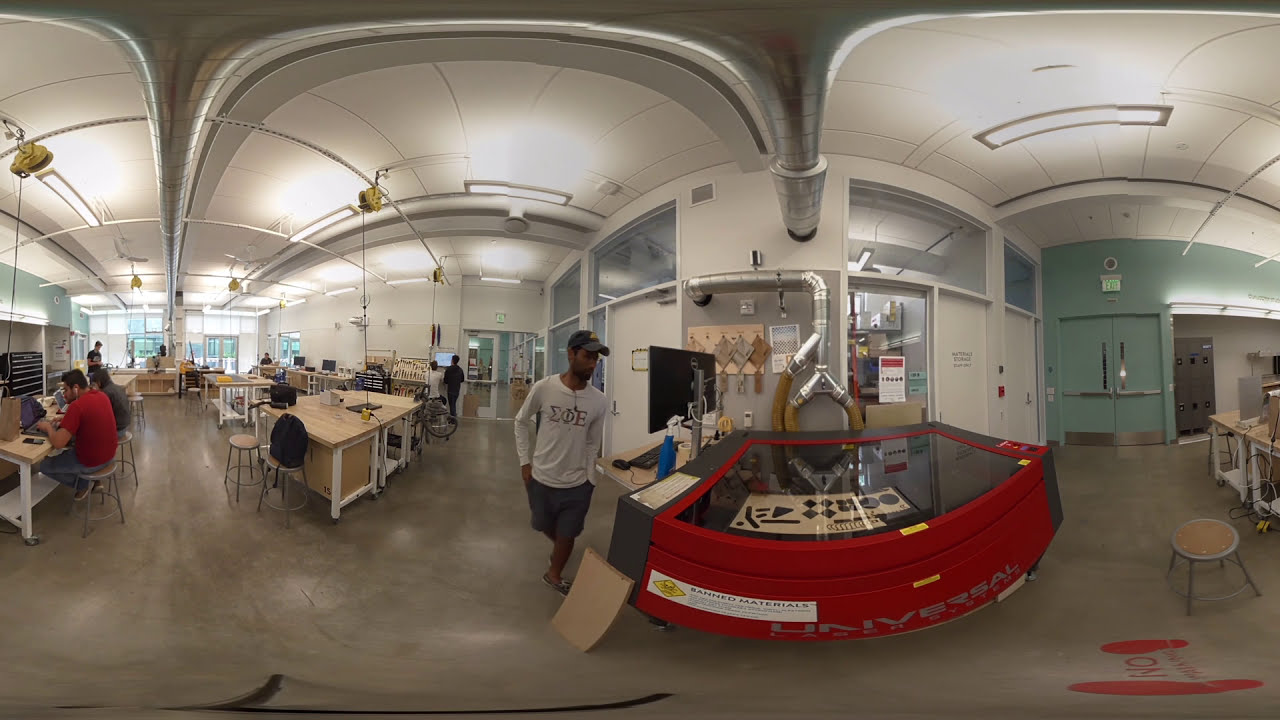In the image, we see the interior of what appears to be a maker lab or fabrication studio, likely within a college setting, given the casual attire of the individuals and the presence of a fraternity shirt with Greek symbols, including Sigma and Epsilon. The large room has a concrete floor, white walls, and a standard white drop ceiling, with visible sections of arched white ceilings adding to the architectural detail. 

Central to the image is a prominent red display labeled "Universal," housing a glass case that contains unknown artifacts. The display is in the center-right of the image. Next to it, a man wearing a white shirt with a logo that possibly says "Zoe," gray shorts, and a gray baseball cap is seen walking, with the back of a computer terminal visible to the slight left, presumably used to control a large CNC laser cutter seen in the room, which cuts medium-density fiberboard (MDF). Ventilation pipes extend from this machine, hinting at its industrial use.

On the left side, people are engaged with their laptops at wooden workbenches, while others are standing and working on various projects. More desks and workbenches with people working are visible along the right side as well, suggesting this is a busy, collaborative space. To the far left and right, multiple doors—some gray and some white—are noticeable, leading to other rooms, with green doors marking an exit on the right. Extension cords are neatly rolled down from the ceiling, emphasizing the room's functional design for various projects and tasks.